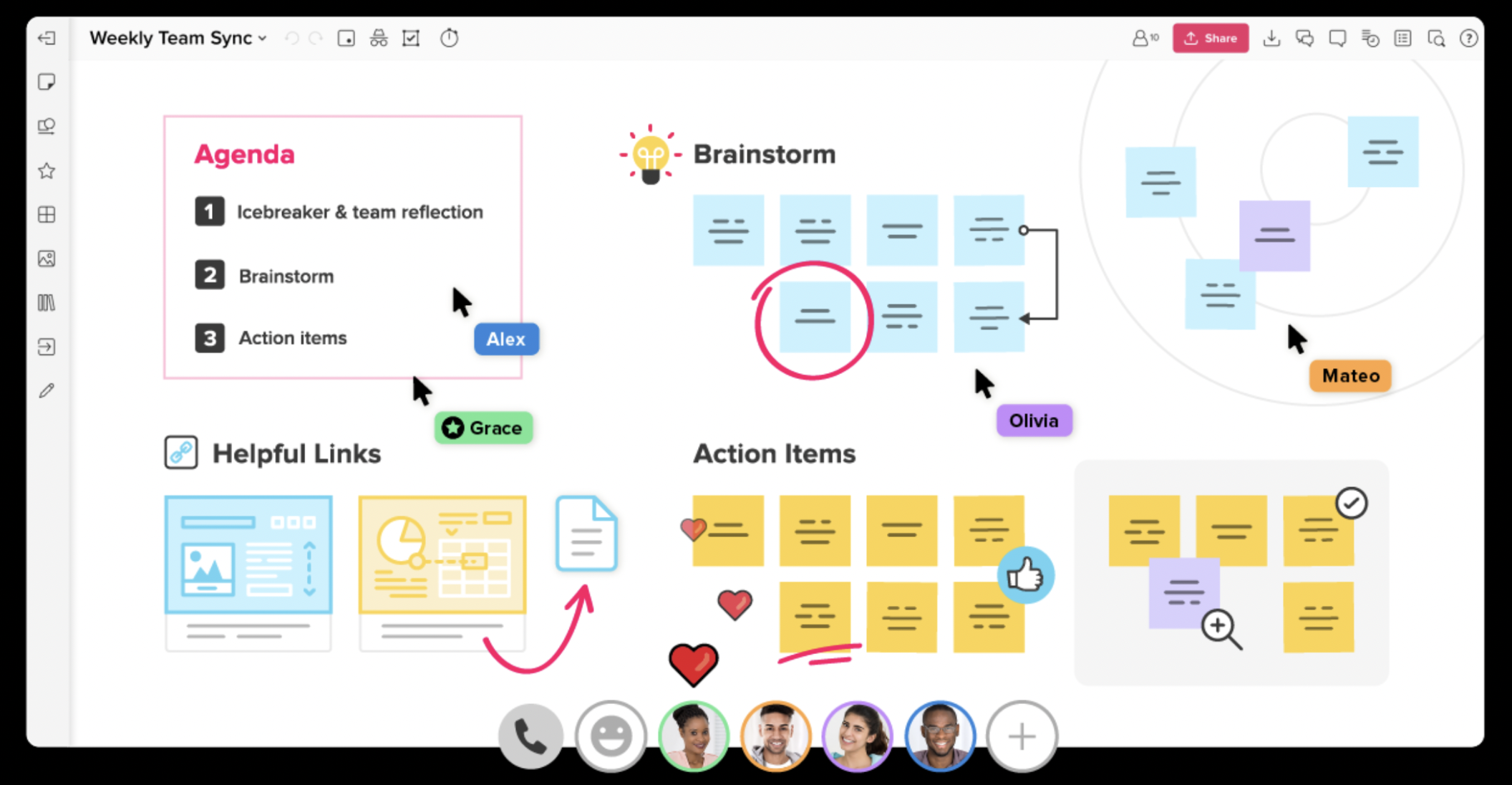The image is a detailed screenshot of a digital bulletin board designed for a weekly team sync meeting. At the top left corner, it prominently displays the title "Weekly Team Sync" along with an agenda boxed in pink, which includes three main items: "1. Icebreaker and Team Reflection," "2. Brainstorm," and "3. Action Items." Below this, there is a section labeled "Helpful Links" accompanied by various icons that resemble reports or documents, highlighted with an upward pointing magenta arrow. 

To the right of this, there are colorful post-it notes: yellow notes under the heading "Action Items" and other notes under the heading "Brainstorm." Notably, the brainstorming section has content encircled in magenta, and the action items section features underlined text in the same color, along with a thumbs-up icon beside one of the items.

At the bottom of the screen, a phone call icon and an emoji menu are visible. Next to these, there are four profile circles, showcasing the faces of team members logged into the meeting: a brown-skinned woman with her profile circled in green, a gray smiley face within a gray circle, and a caramel-skinned man encased in an orange circle. The overall background of the interface is white, with additional colored text boxes and arrows to help guide the viewer's attention. The visual style and layout emphasize the structured and interactive nature of this online meeting tool, facilitating icebreaking, brainstorming, and action planning.